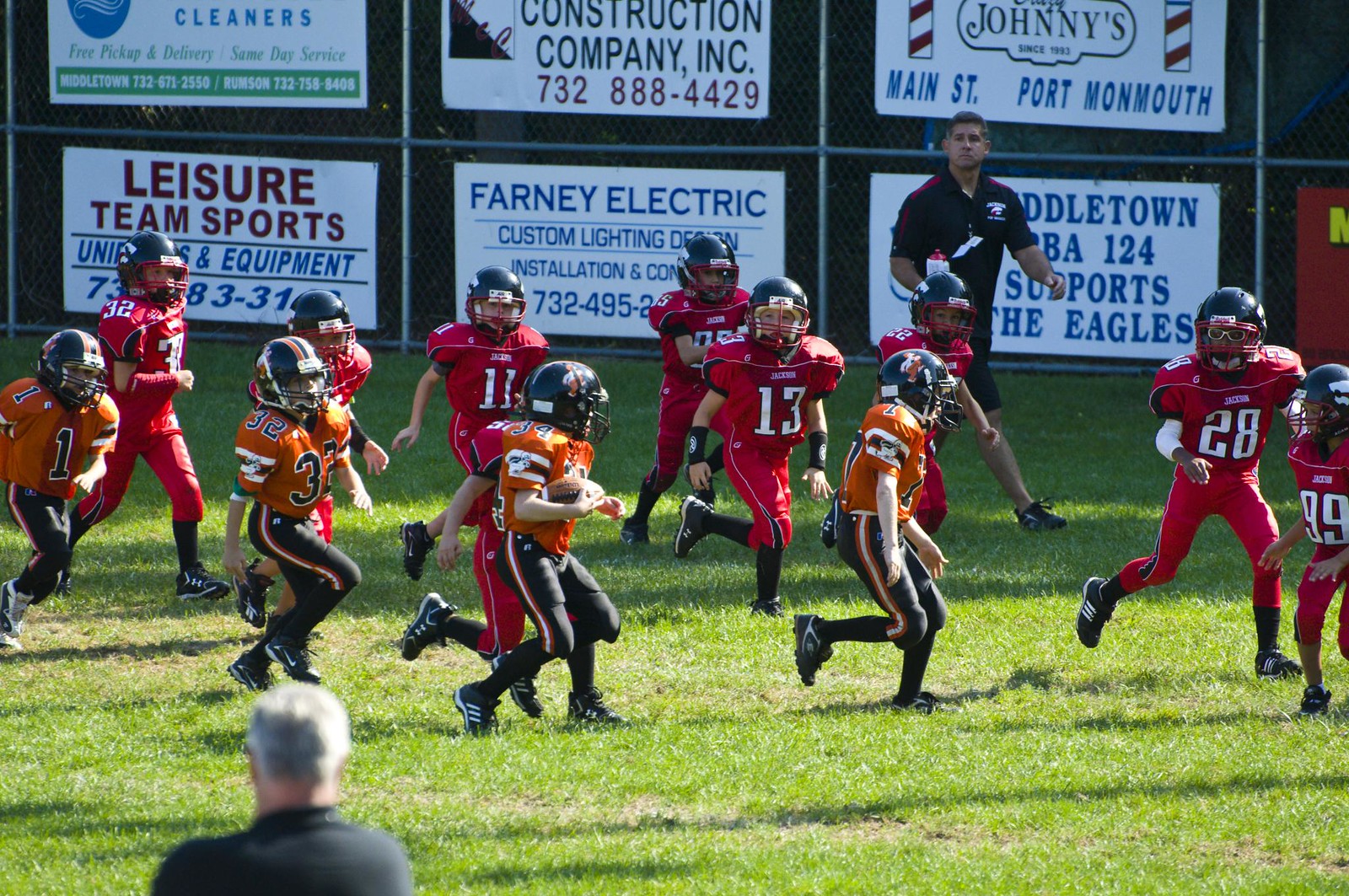The photograph captures a lively youth football game on a grassy field. In the foreground, a player near the center is clutching a football, sprinting while a player from the opposing team prepares to tackle him from behind. The players look no older than 10 years, dressed in red and orange jerseys - some with black or white numbers - and coordinating pants of either black or red. The helmets appear to be a dark blue or black. Off to the sidelines, to the right of center, a coach in a black jersey observes the action, while further behind him, a referee keeps pace with the game. Adding to the atmosphere, a backdrop fence features a series of large rectangular advertisements promoting local businesses like Farney Electric, Leisure Team Sports, and Johnny's among others. The game unfolds under what seems to be pleasant spring weather, with young athletes and the older spectators embodying the community spirit. An older man with gray hair stands in the lower left foreground, watching the game unfold with keen interest.